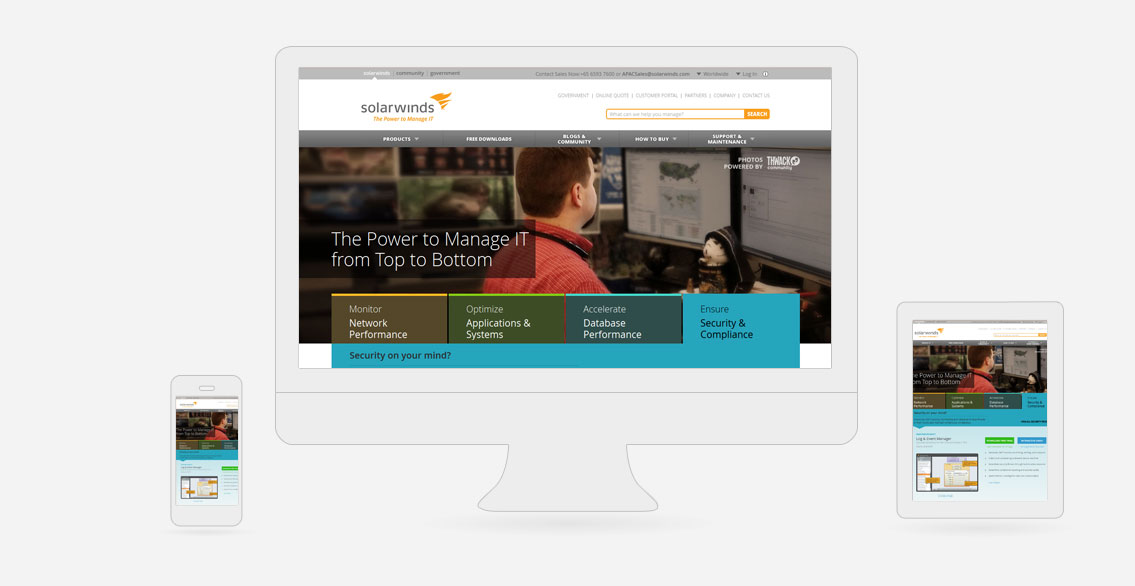This detailed caption describes a screenshot of a website page featuring SolarWinds branding and content:

The screenshot centers around a large gray rectangle depicting a website interface. At the top, a gray horizontal navigation bar spans the width of the page. Situated on the left side of this bar is the SolarWinds logo, featuring the text "SolarWinds" in black accompanied by an orange tornado icon to its right. On the right side, there is text information alongside a search bar highlighted with an orange outline. Adjacent to the search bar is an orange button labeled "Search" in white text.

Beneath the navigation bar, there is a prominent photograph of a man viewed from his right side and back, dressed in a red shirt and engaged with two computer monitors. This photograph encapsulates a typical work environment for managing IT infrastructure.

Towards the bottom left of the page, a black rectangle contains the text "The power to manage IT from top to bottom" in white. Directly below this, a blue rectangle features additional details. Additionally, three small rectangles in brown, green, and blue are aligned at the top of the image, each with white text inside.

The main photograph, along with supplementary content, is depicted within the outline of a computer monitor, accentuated by a gray border. To the left of this image is a smaller representation of the same content displayed on a cell phone screen. On the right side, there is another depiction showing the same content on a tablet screen. These elements together showcase the adaptability and responsiveness of the SolarWinds platform across multiple devices.